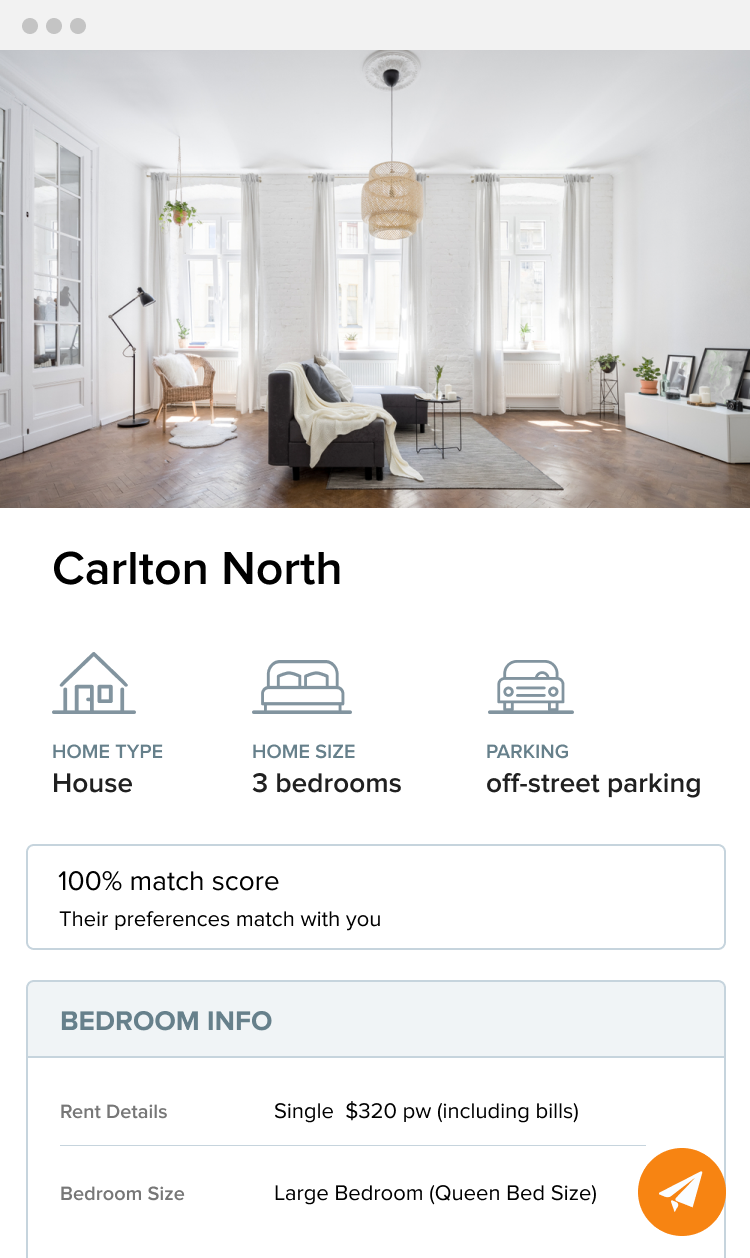A bright and airy living room is showcased at the top of the screenshot, revealing polished wooden floors and pristine white walls that extend up to a white ceiling. The space is illuminated by three large windows, gracefully draped with white curtains, allowing natural light to flood the room. Below the image, the headline reads "Carlton North," indicating the location of this chic house. The property boasts three spacious bedrooms and convenient off-street parking, with a perfect 100% match score for potential renters. The rent details specify a single occupant rate of $320, which includes all bills, for a generously sized bedroom furnished with a queen-size bed. Additional interface elements include an orange circle button with a white paper airplane icon in the bottom right corner and three small gray circles in the upper left corner, possibly representing navigation or additional options.